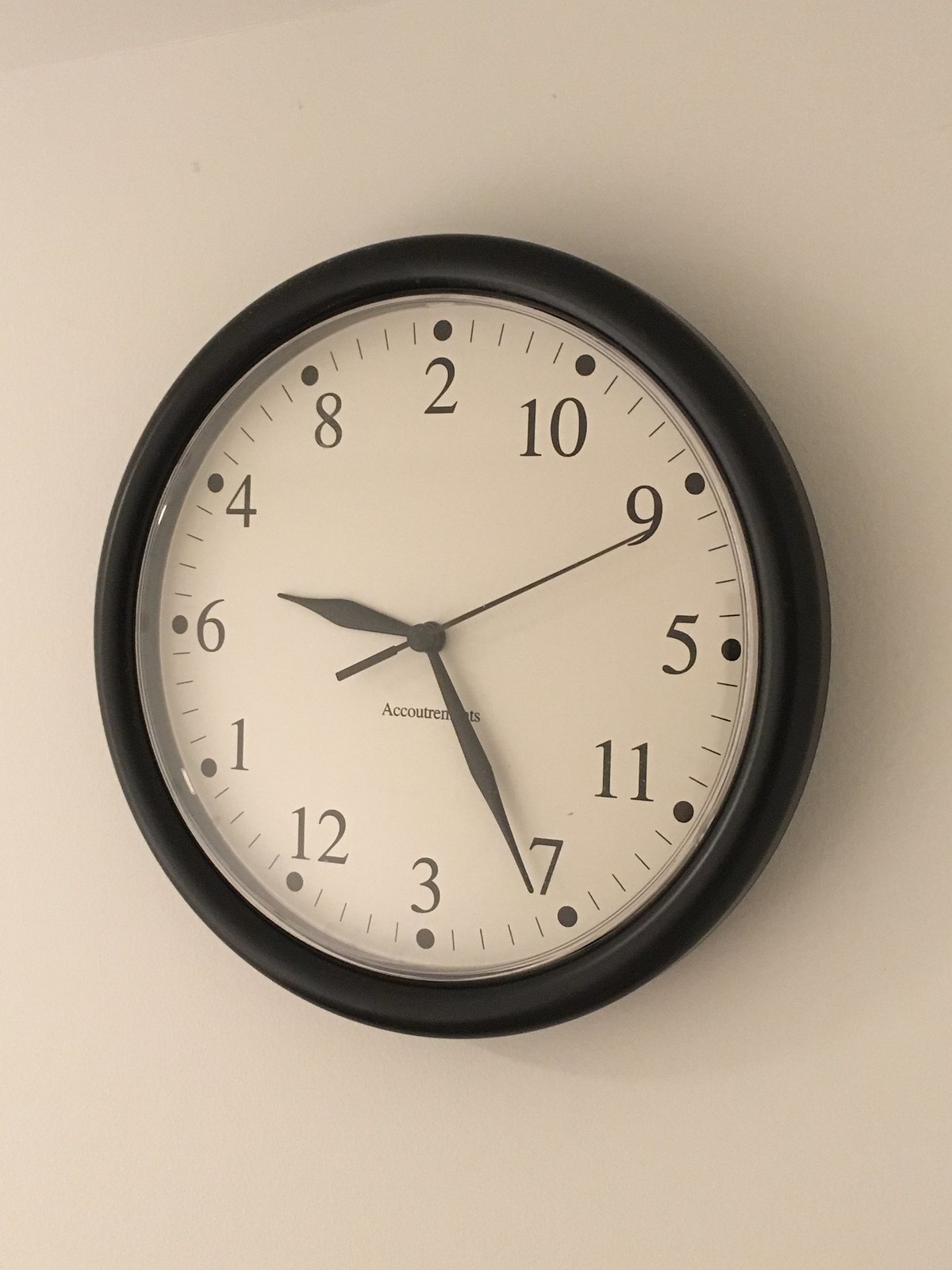The image depicts a unique and artsy wall clock mounted on a plain, beige wall. The clock, which has a black matte frame and a white background, features all twelve numbers arranged in a random, non-sequential order. For instance, where the 12 would normally be positioned, there is a 2; at the 6 position, there is a 3; and at the 9 position, there is a 6. The numbers continue in this jumbled manner, making it a visually intriguing yet potentially confusing piece. The clock has three hands: a long second hand, a minute hand slightly past 7, and an hour hand slightly past 6. The second hand points directly at the 9. The word "accoutrements" is inscribed beneath the hands. The clock casts a slight shadow on the otherwise empty wall, emphasizing its prominence as the sole decorative element.